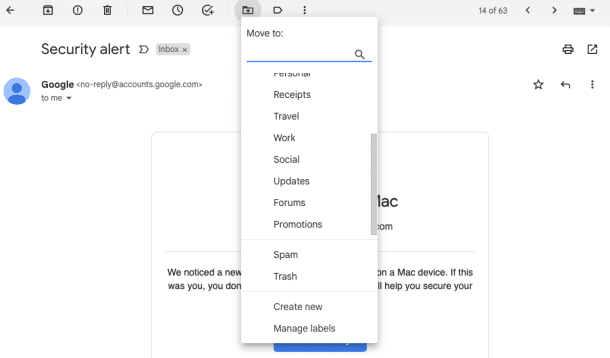The image displays a screenshot of an email interface. At the top of the screen, there is a thin gray bar adorned with various black icons. These icons include a back arrow, a box with an arrow pointing outward, a circle with an exclamation mark inside, a trash can, an envelope, a clock, a circle with a checkmark, a manila folder, a flag-shaped icon, and three dots.

On top of the manila folder icon, there is an open white window with the label "Move to," accompanied by a blue search bar with a magnifying glass icon. The dropdown menu lists options such as Receipts, Travel, Work, Social, Updates, Forms, Promotions, Spam, Trash, Create New, and Manage Labels.

Returning to the gray bar at the top, there is an indicator showing "14 of 63" emails, with adjacent back and forward arrows. Also present is an icon of a keyboard with an arrow pointing down. Beneath these, additional icons include a printer, a box with an outward arrow, a star, a back arrow, and three horizontal lines.

On the right side, within the body of the email, there is a security alert message. The visible part of the subject shows a flag icon, the label "Inbox," and a blue circle with a person icon. The sender is listed as Google, from the email address noreply@accounts.google.com, directed to the reader.

The overlaying "Move to" menu partially obstructs the email's content, revealing only fragments of text. The email seems to be regarding a detected login from a new Mac device. The incomplete message includes phrases like, "we noticed a new on a Mac device," and, "If this was you, you don't..." followed by a partially visible blue box.